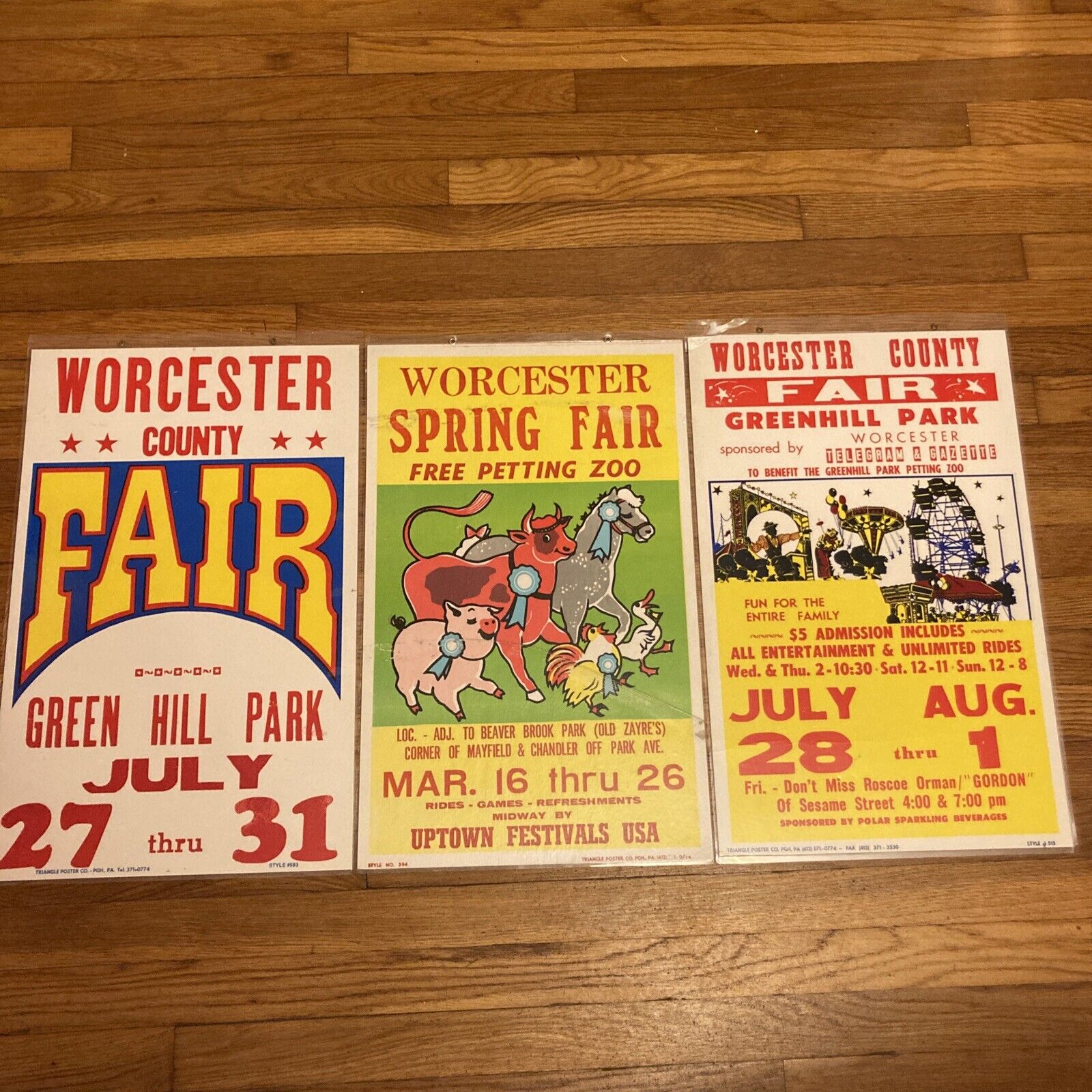The image displays three vintage-styled posters for various Worcester fairs, all mounted against a wooden paneled background. The first poster, featuring a white backdrop with red text, advertises the Worcester County Fair at Green Hill Park, spanning July 27th to 31st, with the word "fair" prominently highlighted in yellow on a blue background. The second poster, with a yellow background and green center, promotes the Worcester Spring Fair, offering a free petting zoo with cartoon depictions of a pig, cow, horse, chicken, and duck, each adorned with blue ribbons except for the duck. This event runs from March 16th to 26th and includes rides, games, refreshments, and a midway by Uptown Festivals USA. The final poster details another Worcester County Fair at Green Hill Park, mentioning sponsorship for the Green Hill Park Petting Zoo, and advertises an array of carnival rides and family entertainment for $5 admission from July 28th to August 1st. All three posters, encased in plastic wrap and slightly spaced apart, rest on a wooden surface with narrow, aged slats, adding a nostalgic feel to the presentation.